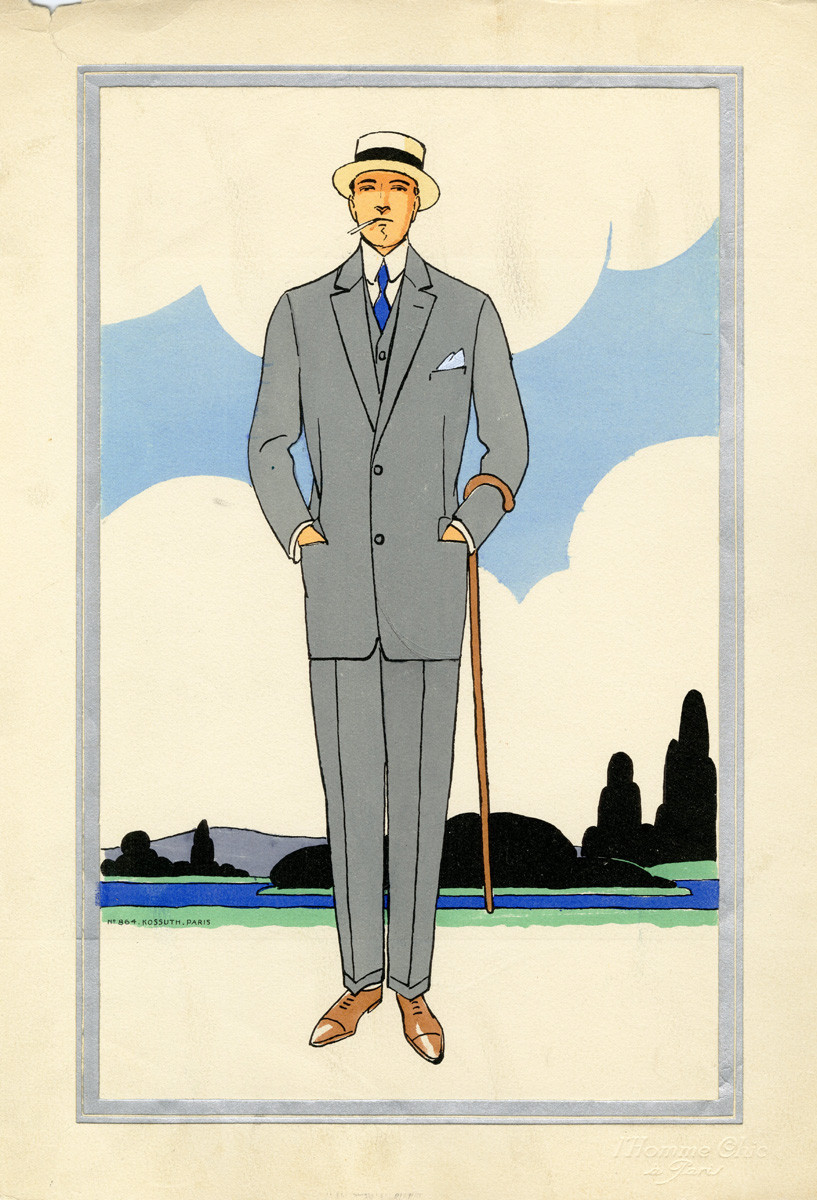This image resembles a vintage cartoon drawing with a striking resemblance to an old-time poster from the 1930s or 1940s. It prominently features a poised Caucasian man standing tall and looking forward. He is professionally dressed in a gray suit that includes a gray vest, a bright blue tie, and a white shirt. Completing his outfit are brown shoes and an off-white hat with black trim. He carries a brown wooden cane strapped around his left arm and has a light blue handkerchief tucked into his breast pocket. Notably, a cigarette hangs from his mouth. 

The background portrays a scenic panorama with beige clouds scattered across a blue sky. The lower part of the image showcases a landscape consisting of black mountains, vivid greenery, and a hint of blue water, all contributing to a naturalistic setting. Black silhouetted trees are sporadically visible, appearing to sprout from a grassy field. The entire composition is framed by a light blue border, with the creamy, bluish-white paper further accentuating the primary colors in the print—gray, white, blue, black, and tan. Overall, the image is a skillfully drawn and visually cohesive representation, blending elements of modern style with a nostalgic touch.